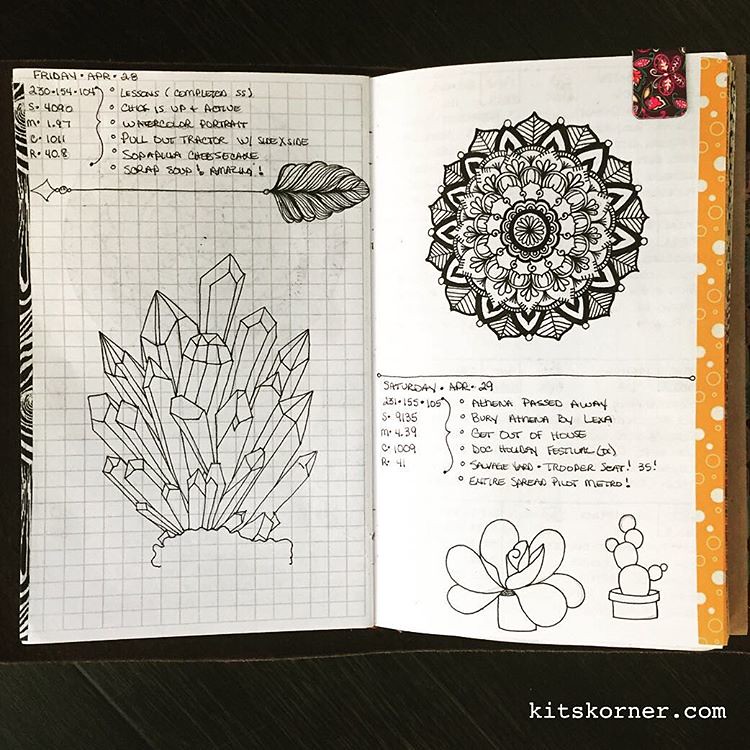The image shows an open scrapbook or artist's notebook with detailed black and white illustrations and text. On the left page, there is a grid pattern adorned with diamond-shaped crystals and leafy or floral drawings. At the top, it says "Friday, April 28th" followed by a list including "Lessons Completed, Watercolor Portrait, Pull Out Tractor, Scrap Soup," and a detailed drawing of quartz crystals below an arrow with a feather. On the right page, against a yellow bubble border, there is a large, fractal or mandala-like flower design at the top, with text reading "Saturday, April 29th, Somebody Passed Away, Bury Athena by Alexa, Get Out of House, Doc Holiday Festival," followed by images of a potted flower and a cactus. The backdrop of the pages is a dark gray striated surface, and the bottom right corner features the website kitscorner.com. A flowery butterfly bookmark with black and red design peeks out from the top.